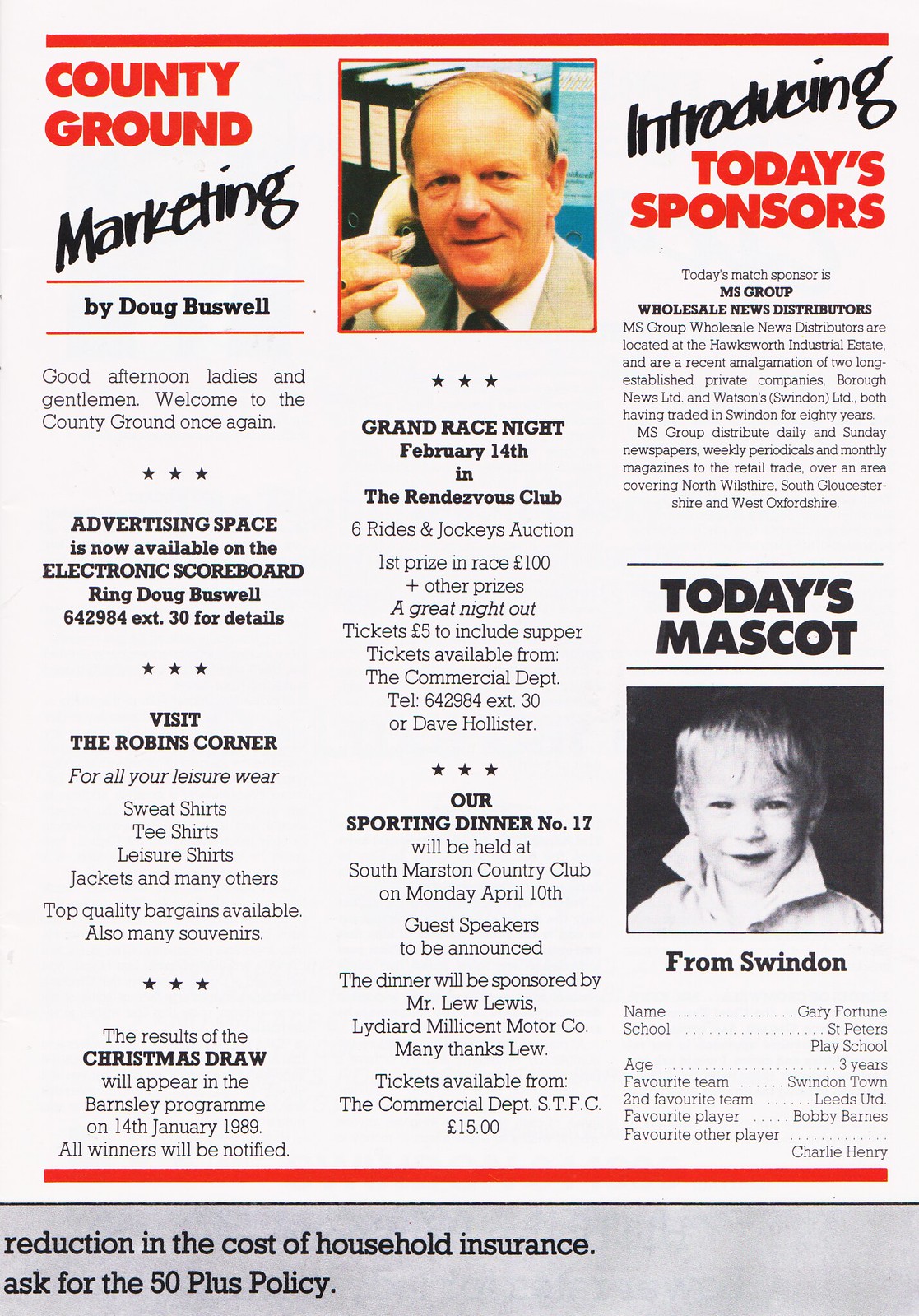This image appears to be a page from a black and white newsletter with red spot color. It is divided into three vertical columns under a thick red line that runs across the top. The left column features the bold red heading "County Ground" at the top, followed by "Marketing" in bold black script. Below this, in smaller black letters, is the name "Doug Buswell." Underneath are several paragraphs of text, interspersed with three asterisks that divide the sections. 

The center column begins with a color photograph of an older man with a short haircut, wearing a gray suit, black tie, and a white collared shirt. He holds an old-fashioned telephone in his right hand and is smiling at the camera, with books visible in the background. Beneath the photograph are paragraphs of text, detailing local events like a grand race night and a sporting dinner, separated by rows of three asterisks.

The right column headline reads "Introducing Today's Sponsors," with "Introducing" in bold black handwriting script and "Today's Sponsors" in bold red capital letters. Below this heading are more articles, including one titled "Today's Mascot" in bold black letters. This section features a black and white photograph of a young boy with short blonde hair, wearing a shirt with the collar up, looking directly at the camera. At the very bottom of the page is a gray border with black print, mentioning a reduction in the cost of household insurance and referencing an unreadable policy number.